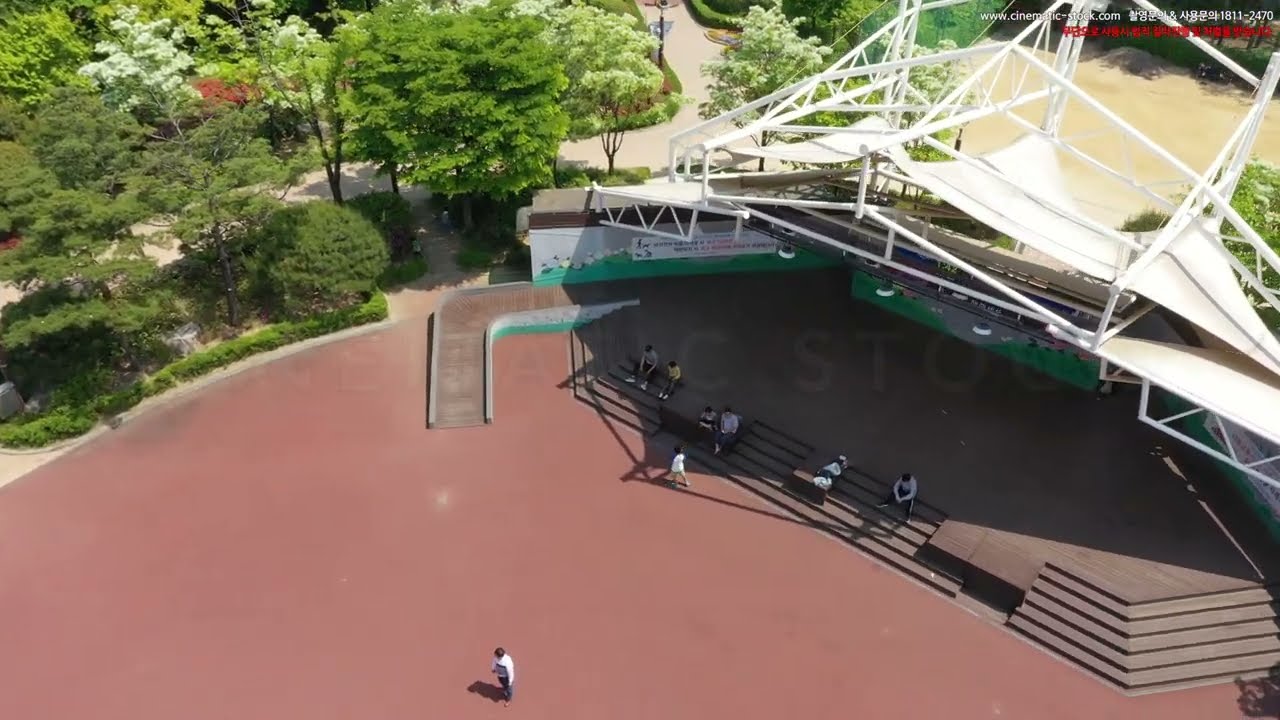This aerial photograph captures an outdoor amphitheater, viewed from what appears to be a high vantage point, possibly a drone. Central to the image is an open, curved area with a reddish-pink surface, possibly dirt or a man-made material. A lone person stands in the middle of this open space. Diagonally to the right of this person, a set of steps leads up to a stage, where several people are seated, enjoying the shade provided by a sail-like covering supported by a metal framework. To the upper left of the amphitheater, a walkway curves around the central area, bordered by trees and bushes, and extends towards the top middle of the photograph. There is a bare spot in the upper left of the image where the surface composition is unclear. Additionally, some text in Korean, along with a URL (www.cinematic-doc.com), appears on the right-hand side of the photograph.